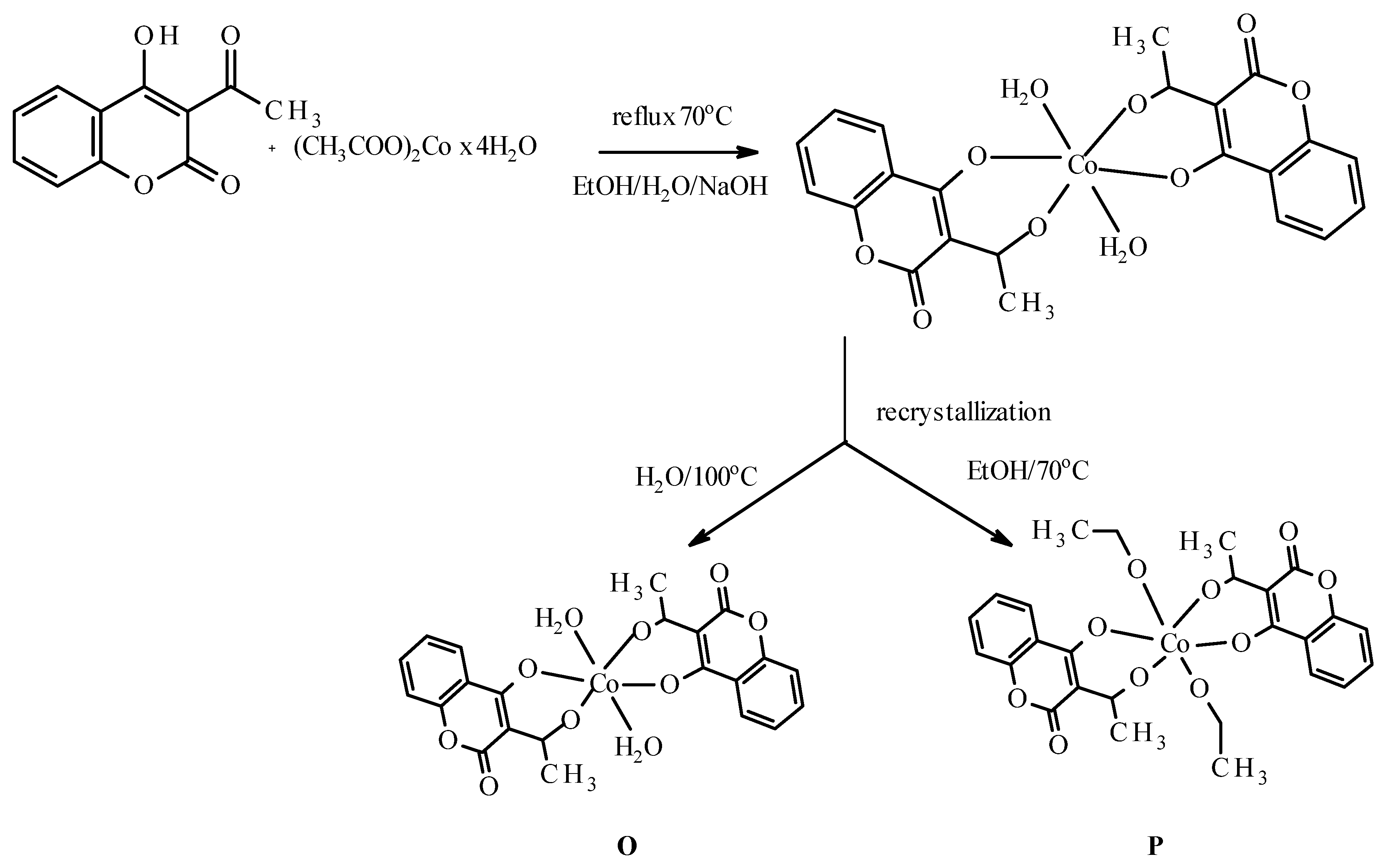The diagram is a detailed representation of an organic chemistry process featuring various chemical formulas and stages. On the left, we see compounds such as OHOCH3 and CH3COO2CO4H2O. In the middle, there's a label "reflux, 70°C" accompanied by chemical notations ETOH/H2O/NaOH, signifying different conditions of the reaction. The diagram on the top right is larger and contributes to the overall process, which involves these organic compounds undergoing a reflux process at 70 degrees Celsius. Following this, the middle part of the diagram indicates a recrystallization phase producing two different compounds. The recrystallization section has two arrows pointing to separate diagrams, each containing some common chemical elements and groupings. At the bottom, these new compounds are labeled, one as "O" and the other as "P." These components include benzene rings and OH groups, drawn out to illustrate the changes occurring at a molecular level through the chemical reactions.